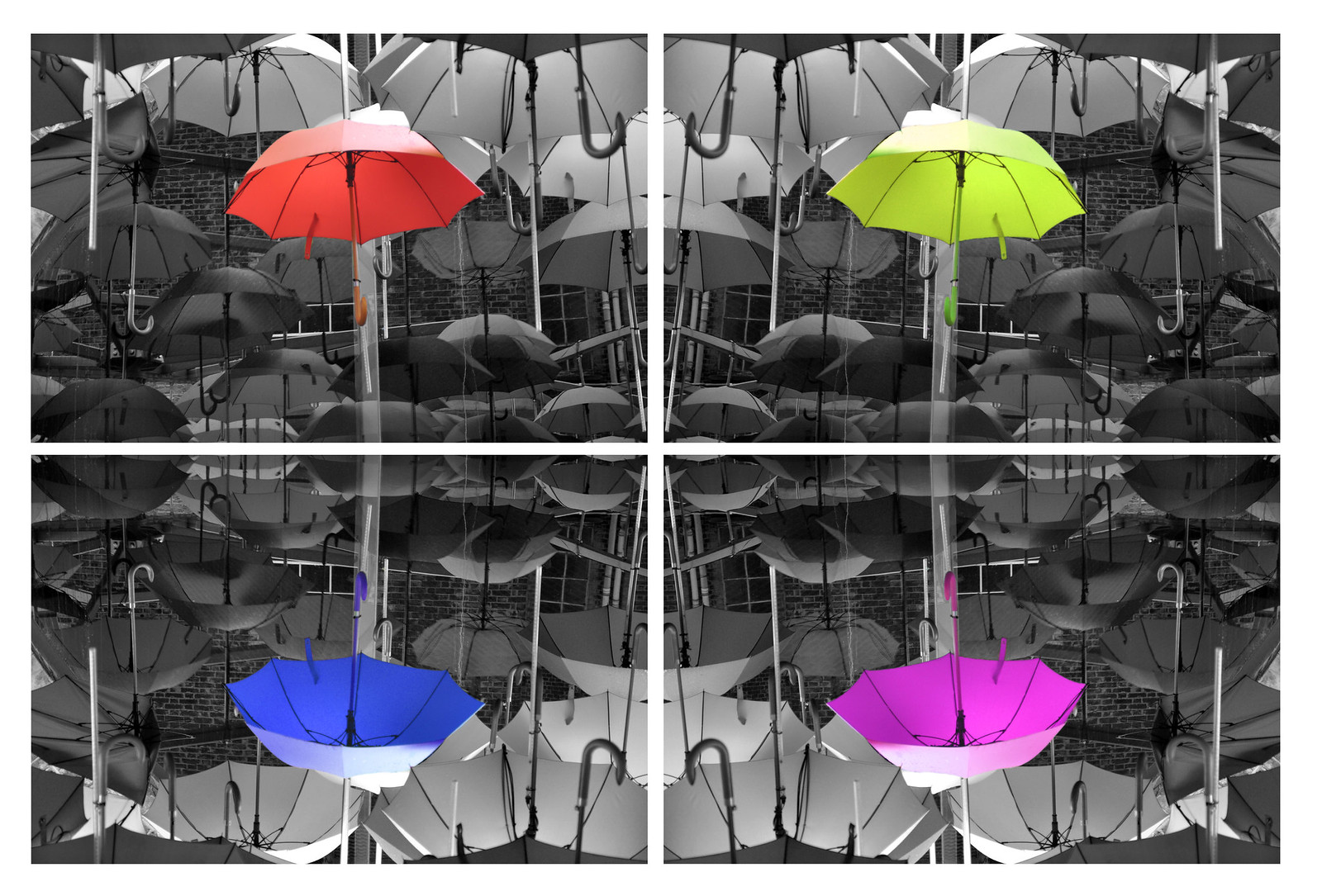This artwork features a composite image divided into four sections by a white border. Each quadrant showcases a vibrant umbrella at its center, set against a monochromatic background of numerous other umbrellas, both right side up and upside down. The top left quadrant displays a red umbrella, the top right showcases a lime green umbrella, the bottom left features a blue umbrella, and the bottom right presents a magenta or purple umbrella. Notably, the red and green umbrellas are open and upright, while the blue and purple ones are inverted with their handles facing up. The overall composition creates a striking contrast between the vividly colored central umbrellas and the black-and-white surrounding ones, emphasizing the artwork's unique and abstract aesthetic.